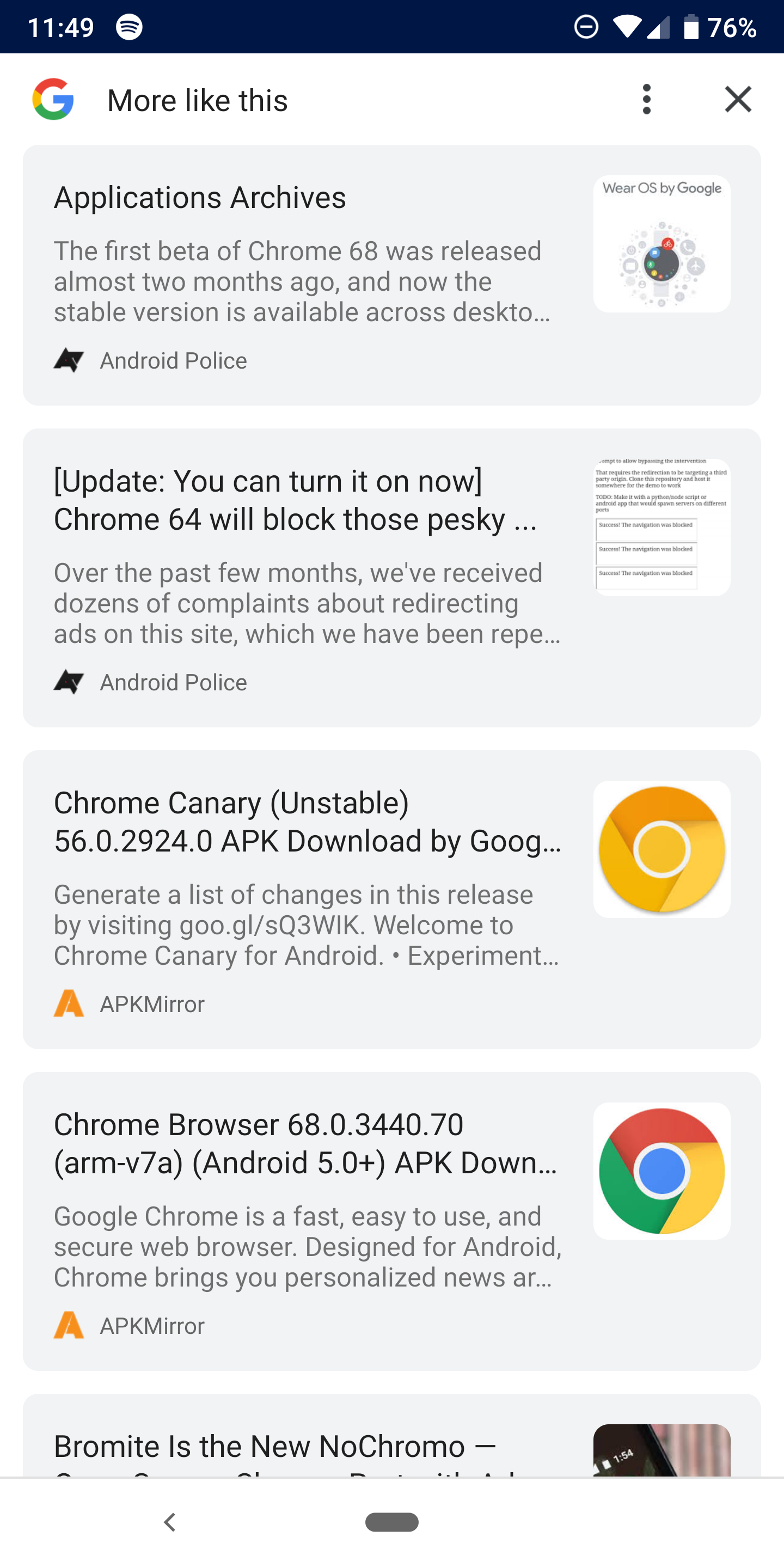The screenshot showcases a Google search results page with the iconic Google logo prominently displayed at the top. Below the search bar, which includes options for refining the search such as "More like this" and a menu denoted by three vertical dots, sits the main body of the search results.

The first result, from "Android Police," involves an article discussing the first beta of Chrome 68, mentioning that its stable version has been released across desktop platforms: "The first beta of Chrome 68 was released almost two months ago, and now the stable version is across desktop..." The snippet includes an update notification in brackets indicating that a feature can now be turned on: "[UPDATE: You can turn it on now] Chrome 64 blocks these pesky..." The text hints at ongoing issues and user complaints regarding redirecting ads on the site.

Below this, a link to an APK download page for Chrome Canary (an unstable version of the browser) is displayed. It includes version details: "Chrome Canary (Unstable) 56.0.294.0 APK download by Google... Generate a list of changes in this release by visiting goo.gl/SQ3WIK." The description also welcomes users to experiment with Google Canary for Android.

Further down is another APK download link for Chrome Browser version 68.0.3400.70 with device compatibility details: "(ARM-v7a) (Android 5.0+) APK download... Google Chrome is a fast, easy to use and secure web browser designed for Android. Chrome brings your personalized new AR..." from APKMirror.

Additionally, the page showcases various icons, notably the standard Google Chrome logo, and a distinct yellow and orange version indicating the Chrome Canary variant. Another result titled "Bromide is the new no Chromo" appears at the very bottom, suggesting an alternative browser.

This comprehensive search result page encapsulates various aspects of the Google Chrome browser ecosystem, including stable releases, beta versions, and related articles, providing a wealth of information for users interested in Chrome updates and downloads.